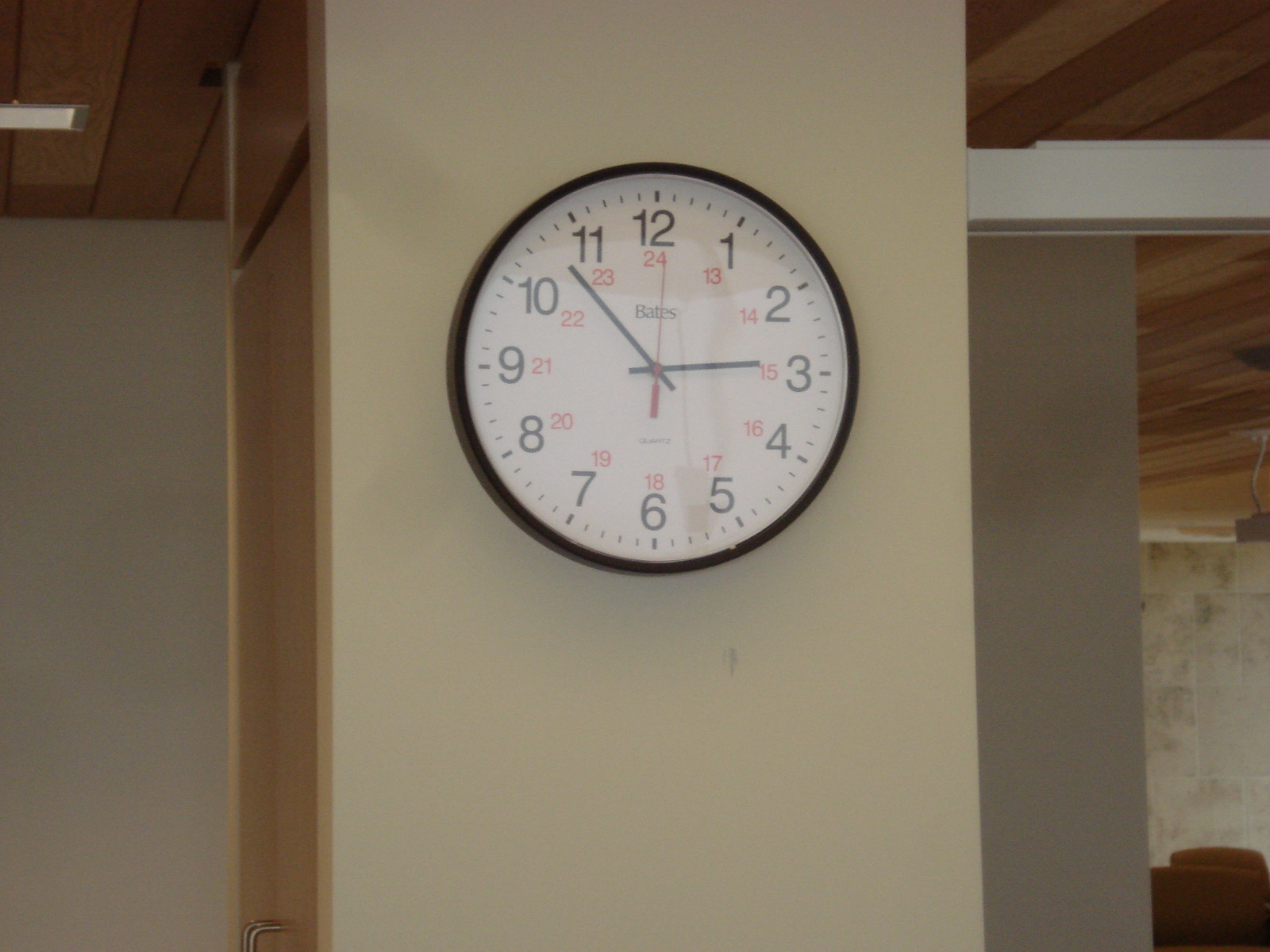This photograph captures a section of an off-white, tan-colored wall adorned with a round clock. The clock features a minimalist design with a black frame, housing a white clock face. The three slender hands are positioned with the hour hand at 3, the minute hand slightly past 1 (approximately 3:08), and the second hand poised at the 1-second mark. The clock is marked with the standard 12-hour format, while an additional set of small red numerals indicates military time (24-hour format). To the left of the clock, a pair of brown double doors adds contrast to the light wall. The image is tightly framed, focusing on this small section of the wall.